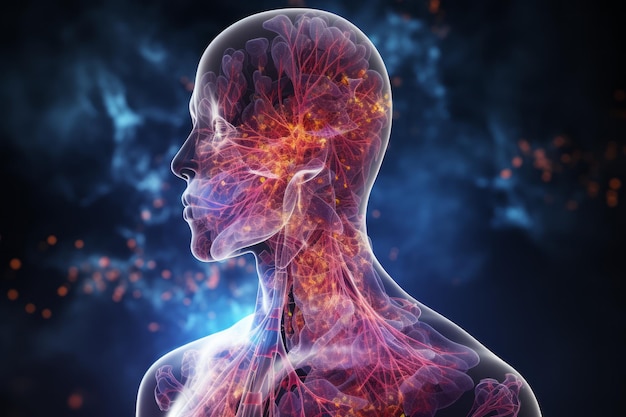The image is a digital, AI-generated artwork featuring a translucent human form, depicted from the shoulders up, turned slightly to the left. The figure is outlined in white, with a bald head devoid of hair, eyebrows, and eyelashes, and all facial features such as eyes, nose, and mouth are present but understated. The inside of the form is filled with intricate, red tentacle-like shapes originating from bright, golden points in the head and neck. These tendrils extend upwards to the head and downwards into the shoulders and torso, giving the interior a complex, almost sci-fi appearance. The background transitions from dark to lighter blue, mottled with white cloud-like formations and scattered with red dots resembling points of light. A bright light illuminates the figure's neck and right shoulder, adding to its futuristic and medical aesthetic.